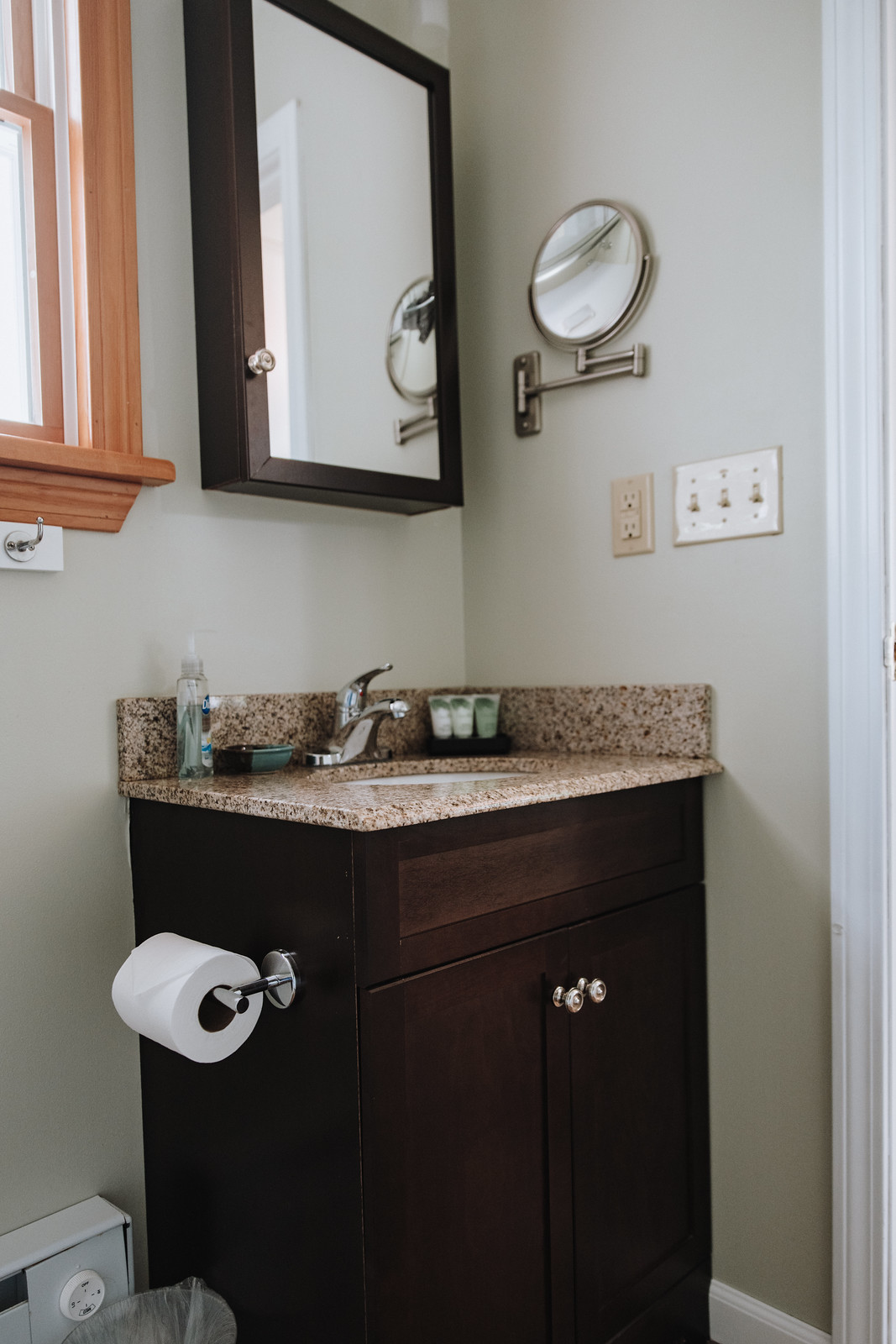This photograph captures a tidy washroom with intricate details. At the center is a dark brown wooden cabinet featuring two white handles. To the left of the cabinet, a silver toilet paper holder with a roll of toilet paper is mounted on the wall. The countertop is a unique brown speckled with black dots, supporting a silver faucet. Nearby, a small black holder contains three tubes, and a clear bottle is placed on the other side of the sink.

The washroom walls are painted white, adorned with a silver light switch panel that includes three switches. Adjacent to the panel, there is a cream-colored electrical outlet. A silver-handled mirror, which can extend from the wall, is positioned above the sink. Another mirror, framed with a dark brown border, is directly in front of the sink. A light windowsill and part of a window are visible, adding natural light to the space.

On the floor beside the cabinet, a garbage bag can be seen, and mounted on the wall is an electric heater, ensuring comfort in the washroom. Each element in the photo contributes to a well-organized and functional bathroom space.